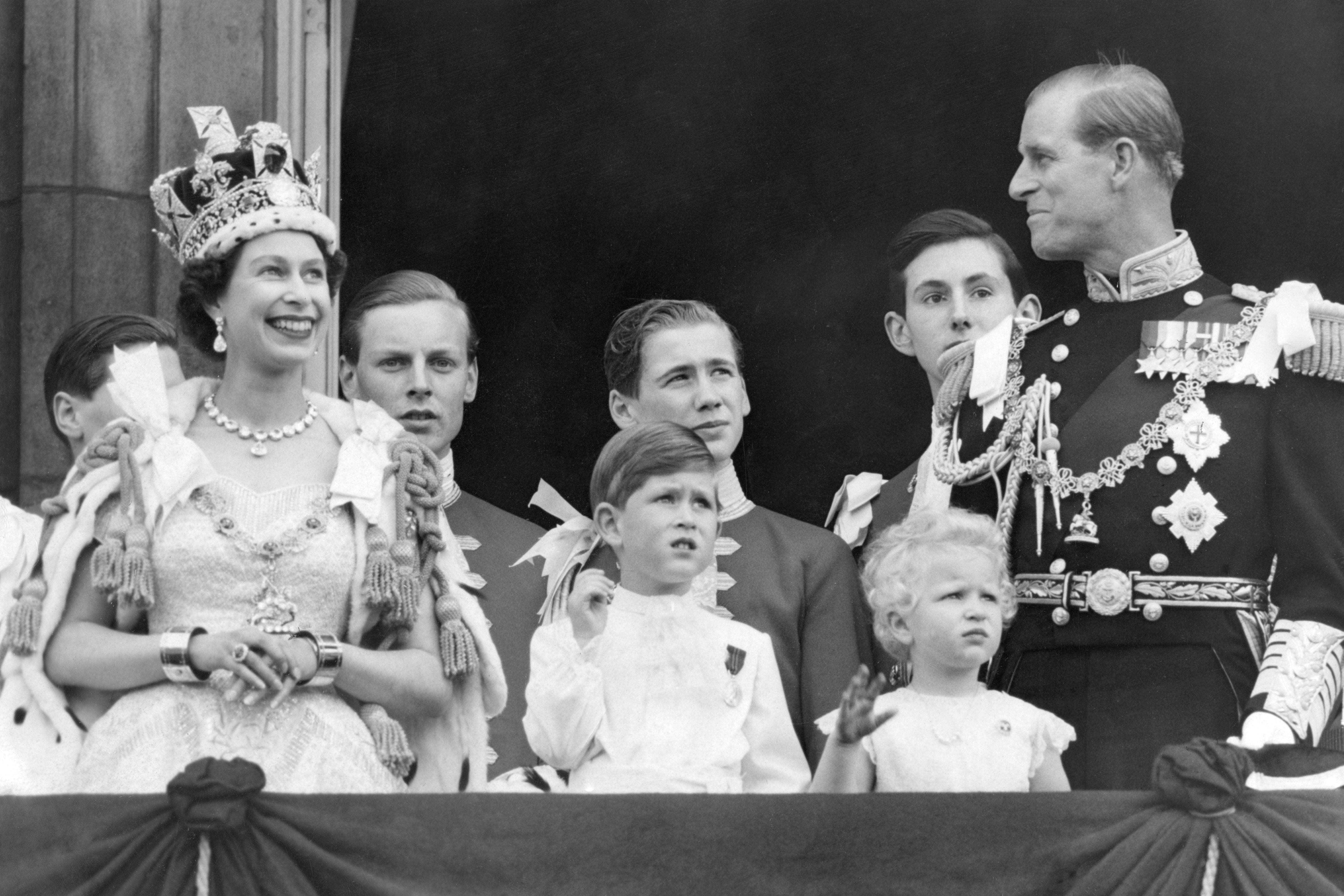In this detailed black and white photograph, a young Queen Elizabeth II, in her 30s, stands regally on a decorated balcony, possibly during her coronation. She is adorned in full ceremonial dress, featuring a large and intricate crown, a prominent gem necklace, earrings, thick bracelets on each wrist, and a large ring. Beside her, Prince Philip is resplendent in his military uniform, complete with fine detailing, thick shoulder pads, a belt with four visible buttons, and an array of medals and honors. Surrounding them are six younger family members, presumably their children and siblings. In the foreground, two small children dressed in white are waving, while in the background, four older children, including Prince Charles, are dressed in more subdued military-like attire. The group’s attention is collectively focused on something tall and unseen in the distance, perhaps a flag. Bunting decorates the balcony, enhancing the celebratory atmosphere of the event, where the royal family observes and acknowledges their subjects below.